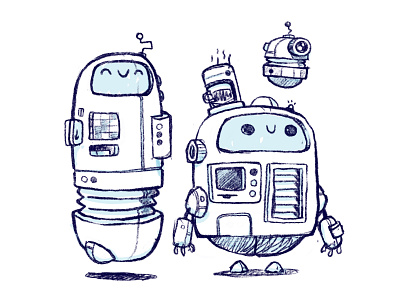The image showcases a whimsical and detailed hand-drawn sketch of three cartoonish robots set against an all-white background, all created with blue ink accents. To the left, a cylindrical robot resembling a pill capsule hovers above the ground with a shadow beneath it. This robot features a face screen with closed eyes and a smiling mouth (or nose), decorative accordion-like ripples in the middle, and a small blue antenna at the top. It also has a latch, buttons, and lights adorning its body.

On the right, there's a shorter, rounder robot with an egg-shaped body. It too is hovering, with detached feet that cast a shadow below. This robot sports a vent panel on its right side, along with several buttons and a small knob on its left. The face screen displays two round black eyes and a smiling face, and protrudes from the top left is an antenna with squiggly lines above it.

Above this round robot floats a tiny robot, also egg-shaped, with one large black eye resembling a camera lens and a small antenna on top. The comprehensive illustration emphasizes the playful and cartoonish nature of these robots, featuring intricate detailing and elements like light blue screens, various buttons, and shadows that enhance their animated, floating appearance.